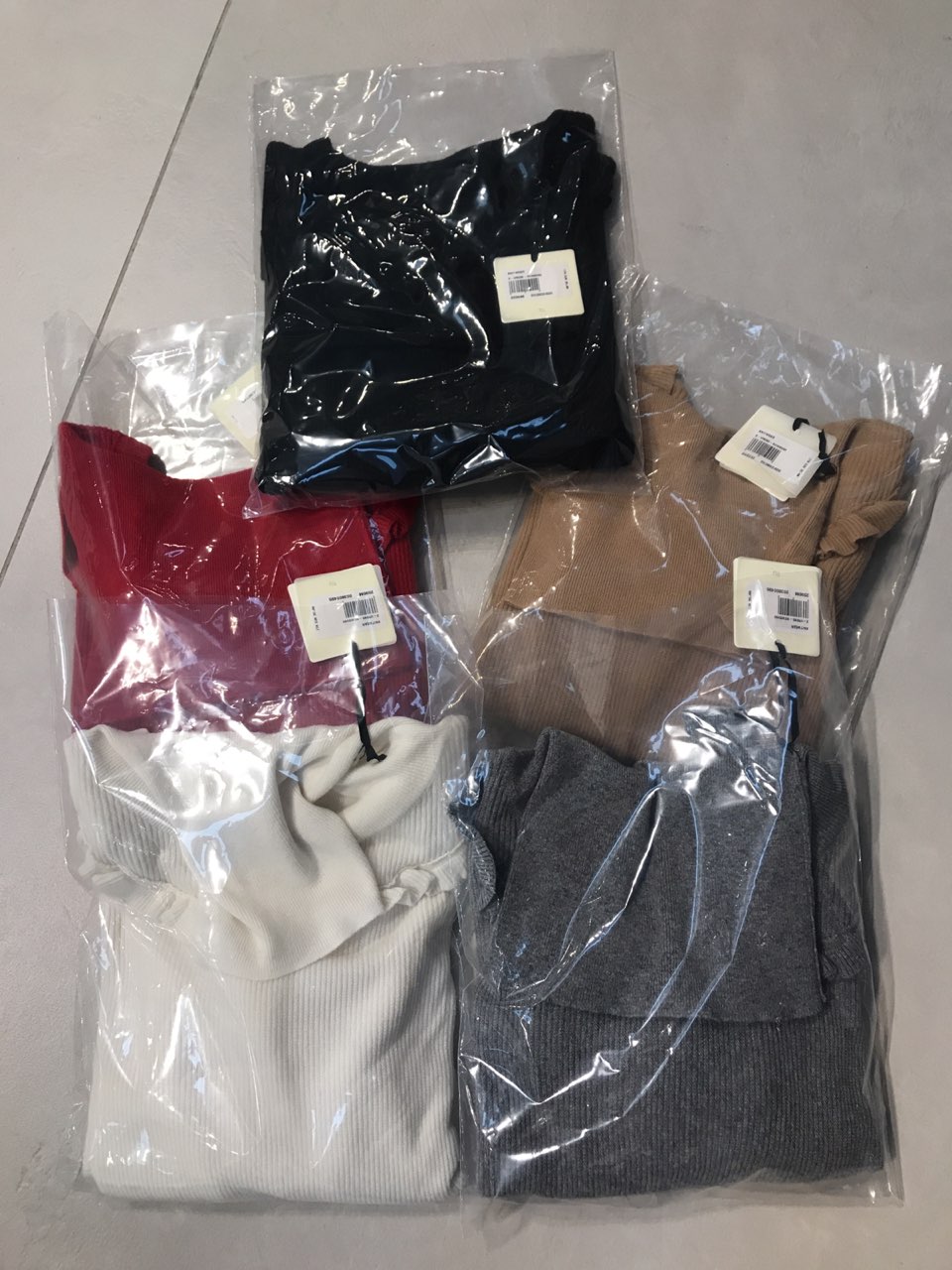The image is a vertically oriented, well-lit photograph with a light gray or white background, likely resembling a tile floor. Central to the image are five folded garments, each sealed in a rectangular plastic bag with beige tags that include barcodes. The garments vary in color and are neatly organized. At the top is a black garment, potentially a sweater or scarf. The top left of the image shows a red garment, while the top right reveals a light brown or camel-colored piece, possibly a turtleneck. On the bottom left, there's a white or off-white garment, which also looks like a turtleneck. Finally, the bottom right features a dark gray item, folded similarly. Each bag appears to be around five inches high and four inches wide, preserving the organized presentation of the clothing items.